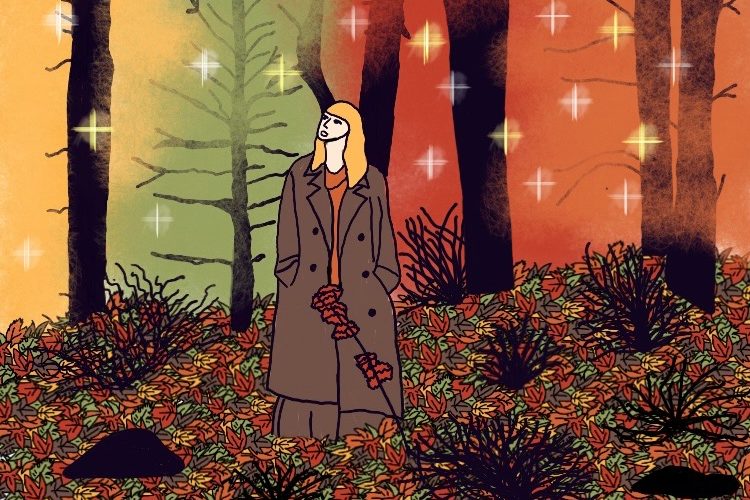The image depicts a hand-drawn illustration of a white woman with long blonde hair, standing in the middle of a forest. She is wearing a large, oversized brown trench coat with her hands tucked into the coat's pockets, complemented by brown pants beneath. The background showcases an autumnal scene with several bare trees, their black trunks surrounded by a carpet of multicolored leaves in shades of red, green, yellow, and brown, along with some black bushes and stones. The woman is looking upward, imparting a thoughtful, serene expression. Additionally, there's a single red flower standing out among the foliage. The sky behind her features a gradient of glowing colors including yellow, green, orange, and red. Various plus-shaped stars in yellow, white, and blue add a whimsical touch to the scenery, further enhanced by sparkles scattered in the air. This piece is executed in a cartoon-esque style with pastel colors, lending it a soft, dreamy quality.